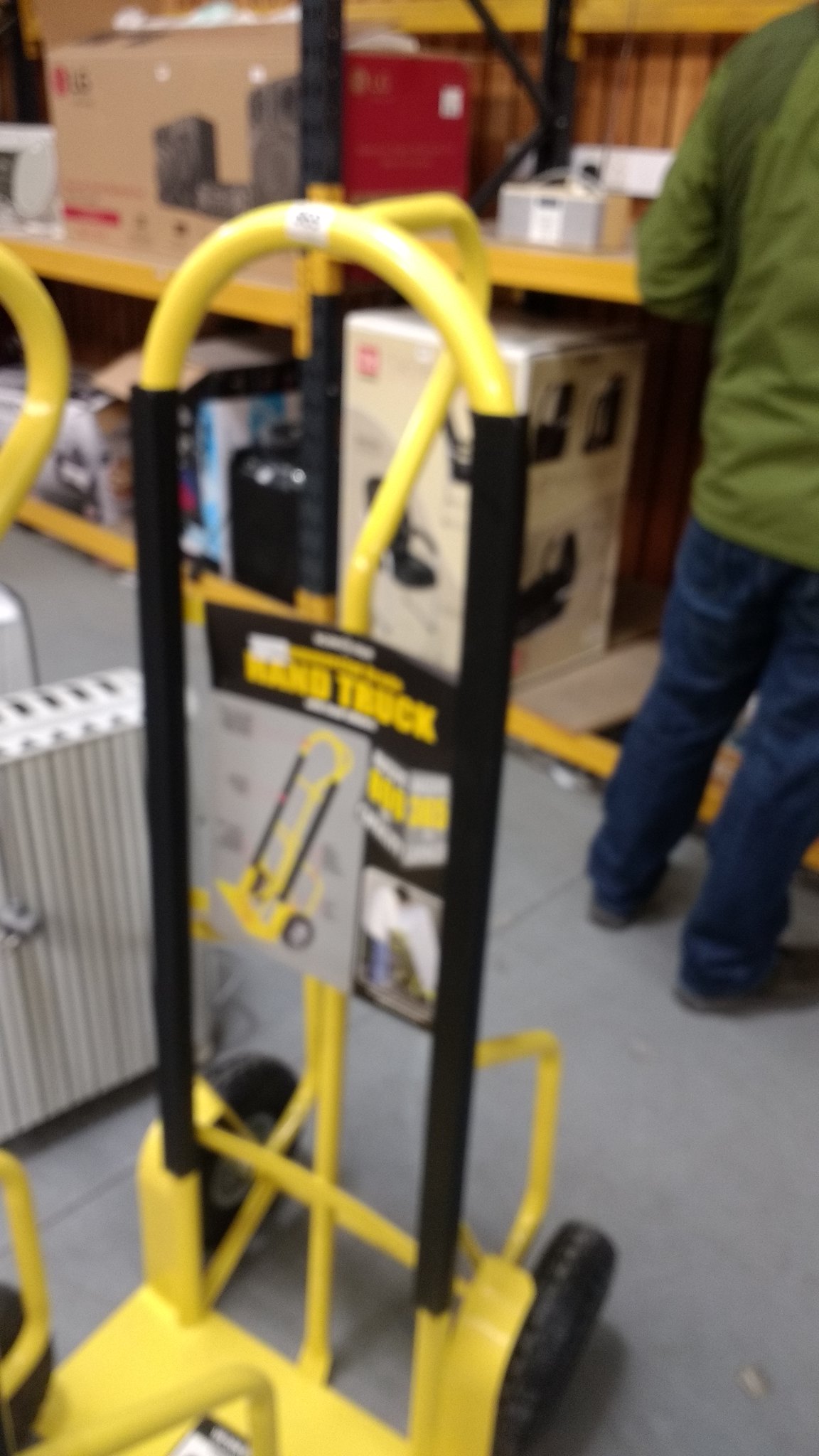The photograph, although slightly blurry, appears to be taken inside a hardware store, possibly a Home Depot or Lowe's. The background features shelving stocked with various cardboard boxes. Prominently on display is a box that seems to contain a stereo system, possibly an LG surround sound set. Other boxes, including a large white rectangular one, can be seen on the bottom row of the shelving. In the upper right portion of the image, there is a person with their back to the camera, wearing a green shirt and blue jeans. In the foreground, to the bottom left, a metal dolly with a yellow base, black wheels, and a yellow handle with black grips and holes is visible. This dolly appears to have a black grip tape on the base, likely to secure items during transport.